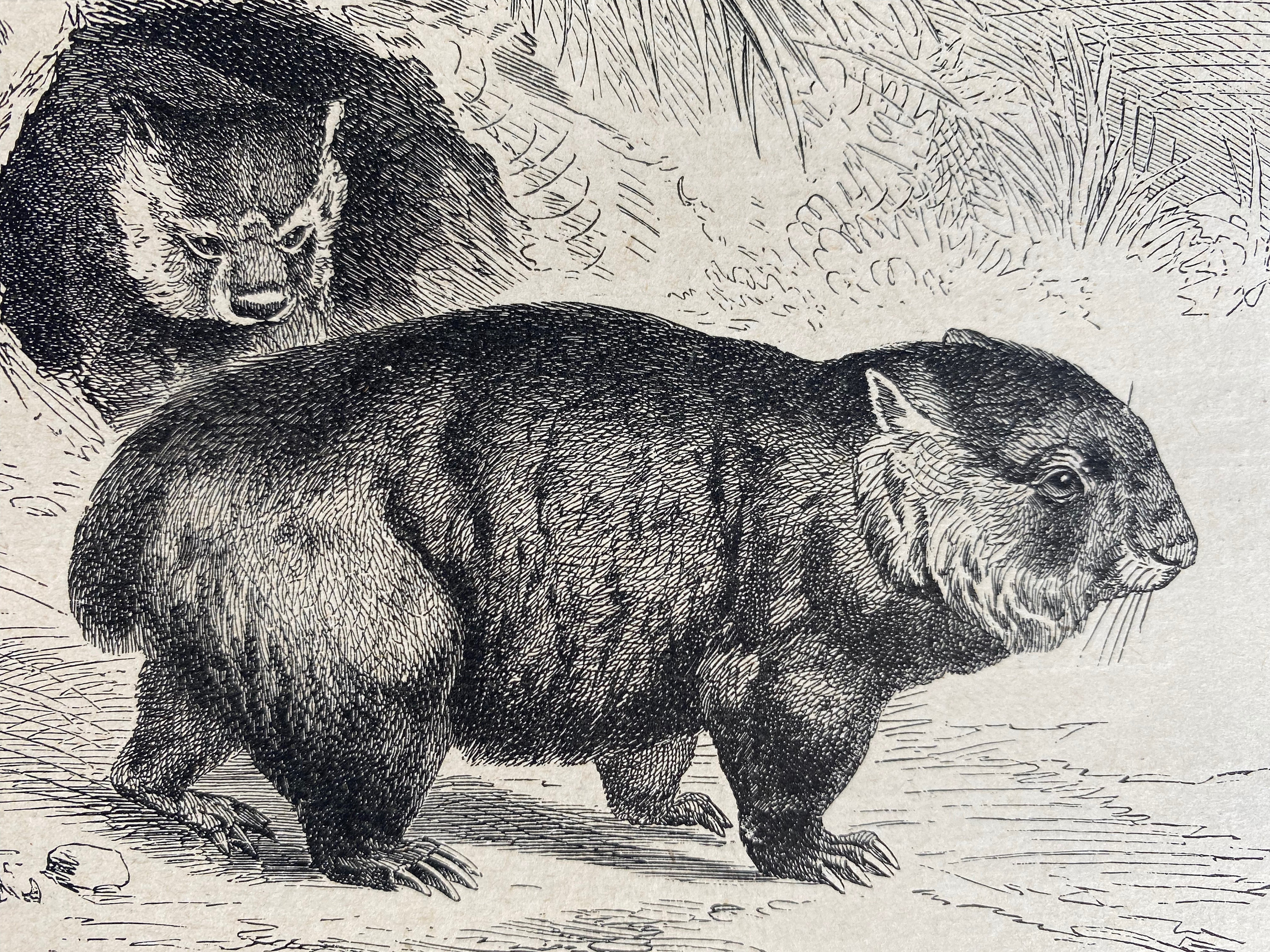This is an antique-looking pen and ink drawing, rendered entirely in black and white. The illustration prominently features a wombat-like mammal walking toward the right, with its whole body visible and its head partially turned, showing its open eye, short pointy ears, and small fluffy tail. Its four paws have sharp claws, adding to its distinct features. In the top left corner of the image, another wombat-like creature appears, showing only its head, seemingly scowling at the main figure. The background is filled with intricate, sketched-out foliage that includes hints of grass and plants, enhancing the scene’s naturalistic element. This unsigned piece captures a detailed and expressive portrayal of these animals in their environment.